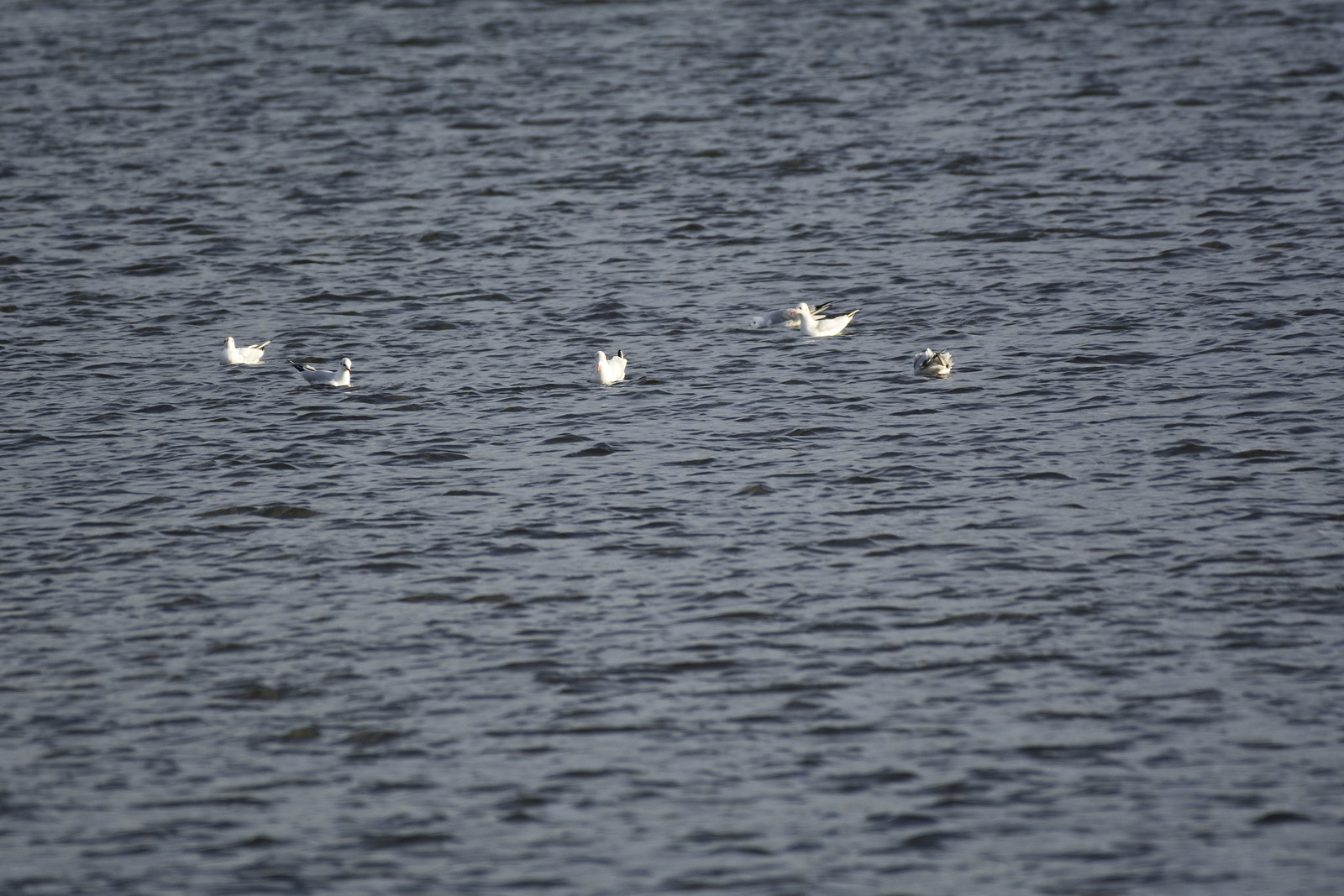The photograph captures a group of five birds floating on the surface of a vast body of rippled, grayish water. The image is slightly out of focus and taken from a considerable distance, making it difficult to discern fine details. The birds are white with gray backs and wings, likely a species of gull, featuring dark beaks and possibly dark feathers in their tails. They are positioned in a rough line near the center of the photo, each facing in different directions. The water around them is characterized by numerous small waves, appearing as gray lines where shadows form. There are no other creatures or man-made objects visible, and the scene is bathed in natural daylight.